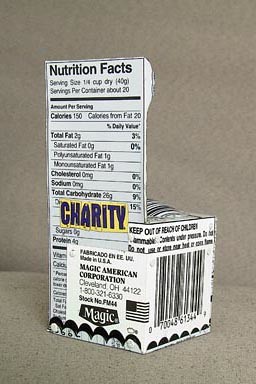On a brown background with a pattern of black dots, the scene captures several important details. On the right side, there is a barcode labeled "7004861344." At the top of the image, a warning reads "Keep out of reach of children." In the bottom left corner, the manufacturing details state "Fabricado en..." and continue with "Made in USA, Magic American Corporation, Cleveland, Ohio, 44122, 1-800-321-630." Near this information, there is an American flag. 

Additionally, there is a nutrition label indicating the following: "Nutrition Facts: serving size: 1/4 cup dry (40 grams), servings per container: about 20, calories: 150, calories from fat: 20, total fat: 2 grams, cholesterol: 0 mg, sodium: 0 mg, total carbohydrate: 25 grams." 

A prominent yellow rectangle with blue text across it reads "Charity." 

Overall, the scene blends critical product information, nutrition details, and a notable callout to "charity," all set against a distinctively patterned brown background.